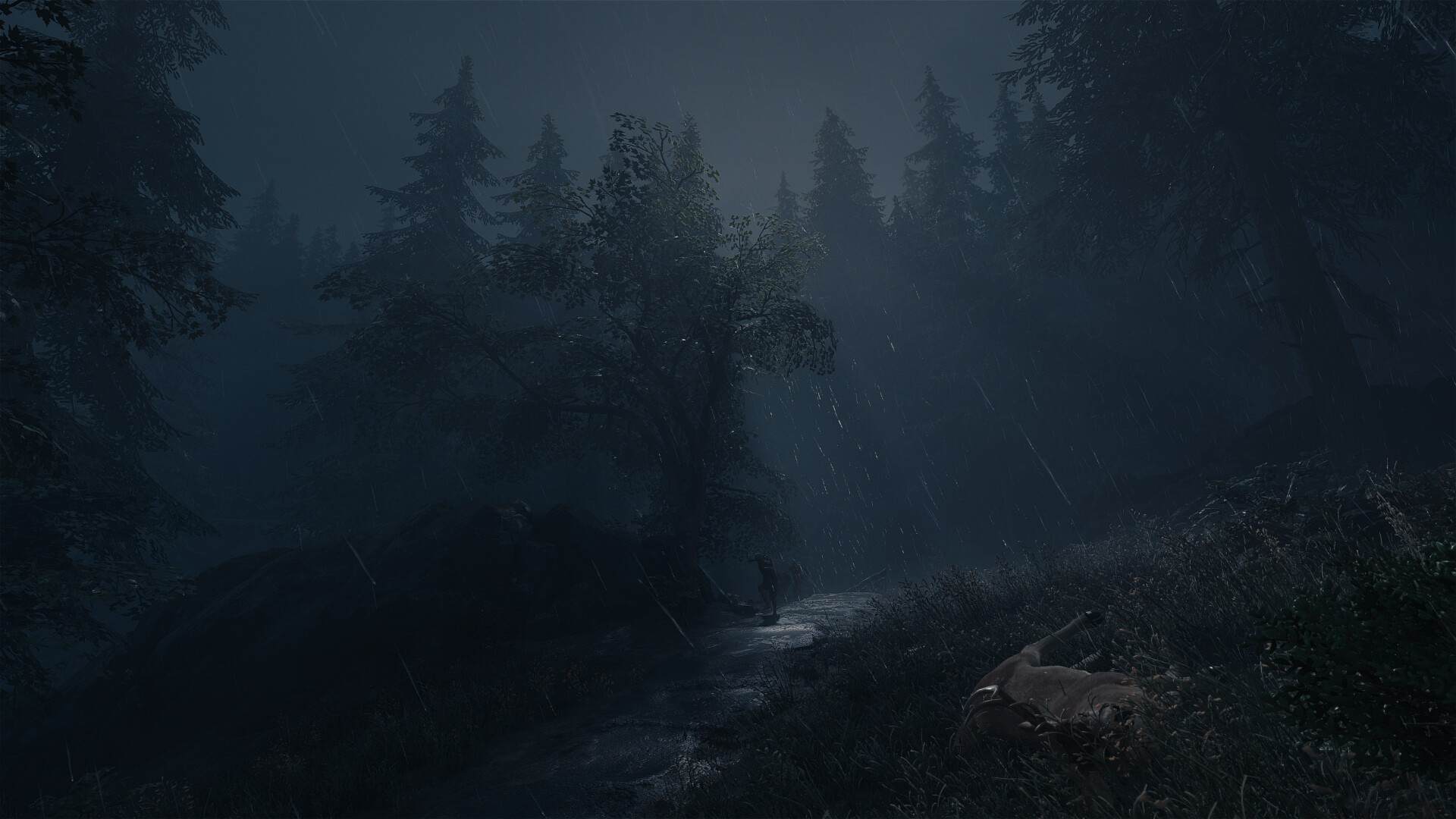The image captures a somber, rainy night in a dense forest. The dark, almost pitch-black sky is briefly interrupted by a small sliver of moonlight that faintly illuminates a muddy dirt road. Towering trees loom over the scene, their forms barely discernible against the inky backdrop. Amidst the obscurity, a dark brown animal, possibly a deer, lies motionless on the road, seemingly injured or deceased. The relentless rain pours down, creating a sense of melancholy and adding to the eerie, desolate atmosphere.